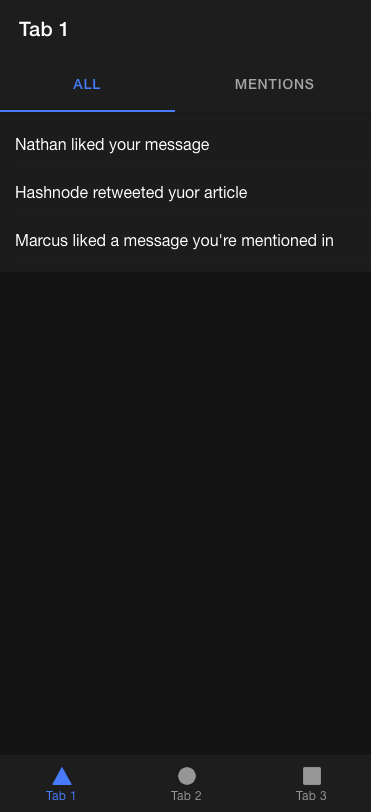Here is a cleaned-up and detailed version of the caption based on the description:

"Screenshot depicting a notification tab on a mobile device. The tab labeled 'All' shows various interactions: 'Nathan liked your message,' 'Hashnode retweeted your article,' 'Marcus liked the message you mentioned.' The interface features a predominantly black background, adding contrast to the white text of the notifications. The layout and functionality of the tab are unclear, and the specific type of device (iPhone or Android) is not specified."